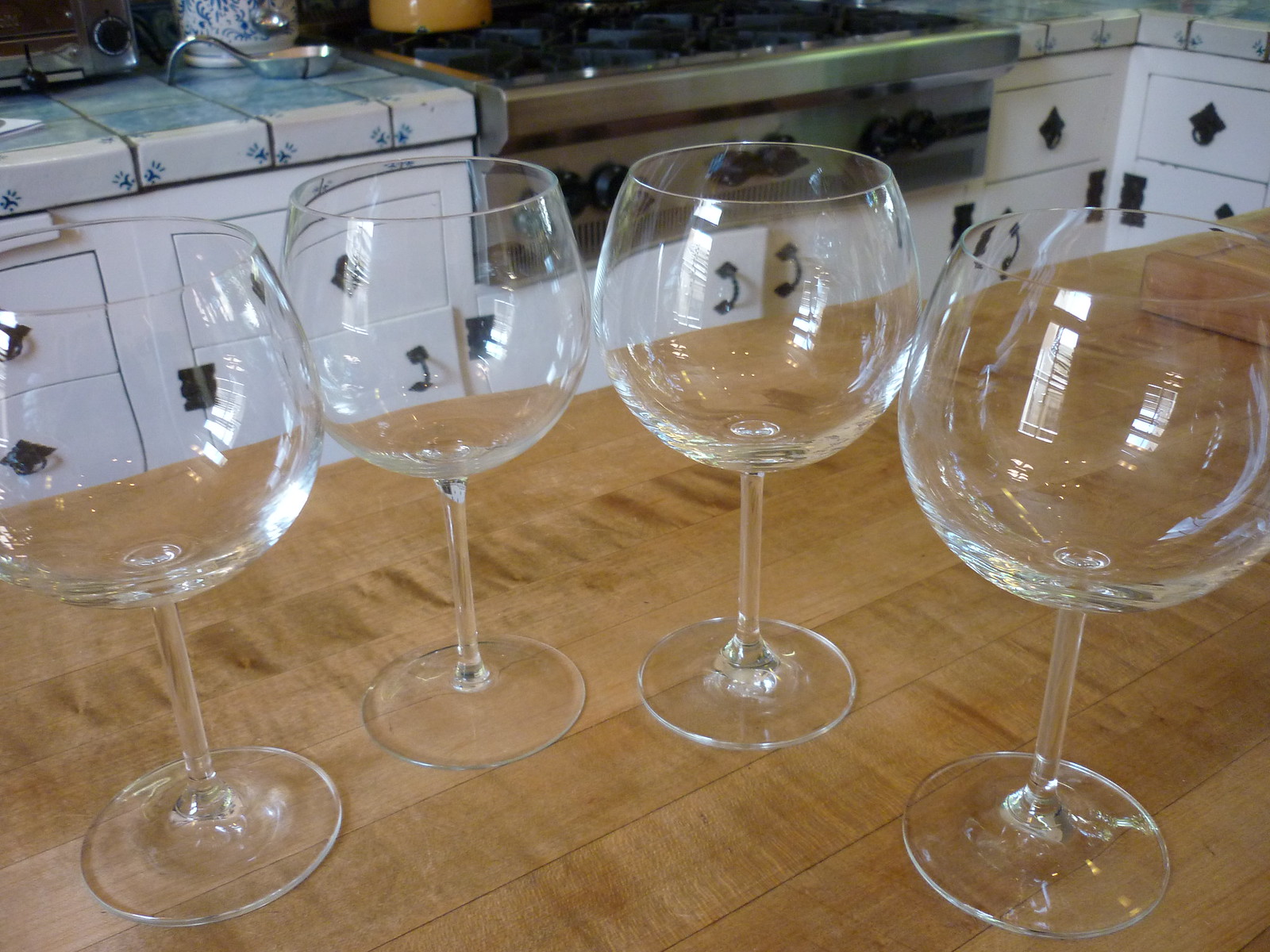This detailed color photo showcases a pristine kitchen scene. In the foreground, four clean and empty glass wine goblets are arranged in a semi-circle on a wooden butcher block countertop. Behind them, a backdrop reveals white cabinets adorned with black handles and a white tile countertop accented by blue floral designs in the corners. The kitchen also features a silver gas stovetop with black knobs and a black grate over the burners, along with a silver spoon rest and an orange enamelware piece chipped to reveal the underlying black iron. Additional elements include a crock and the corner of a toaster oven to the left of the cooktop, lending a lived-in feel while maintaining overall cleanliness. The countertop extends a short distance before turning at a 90-degree angle in the upper right corner, maintaining the uncluttered aesthetic of this well-organized kitchen.